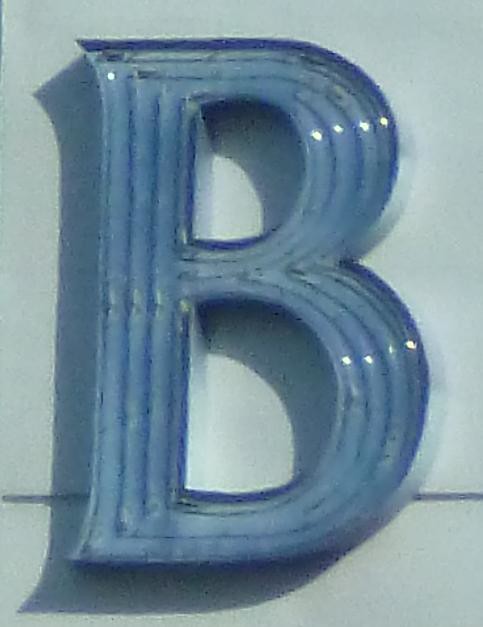This is a close-up image of a large letter "B" displayed on the side of a storefront building. The building itself is constructed from gray stone, providing a neutral backdrop for the prominent letter "B." The "B" is quite large and painted in a light blue color, making it stand out against the gray stone. The design of the "B" incorporates several overlapping lines, creating the illusion of four "B"s nested within each other. Below the light blue "B," there is a dark line that runs almost horizontally near the bottom part of the building. This line appears to be an architectural detail of the building. The photograph seems to be taken during the daytime, as sunlight is clearly visible shining upon the "B," casting a slight shadow below it. This shadow suggests that the sun is positioned above, enhancing the three-dimensional appearance of the letter.